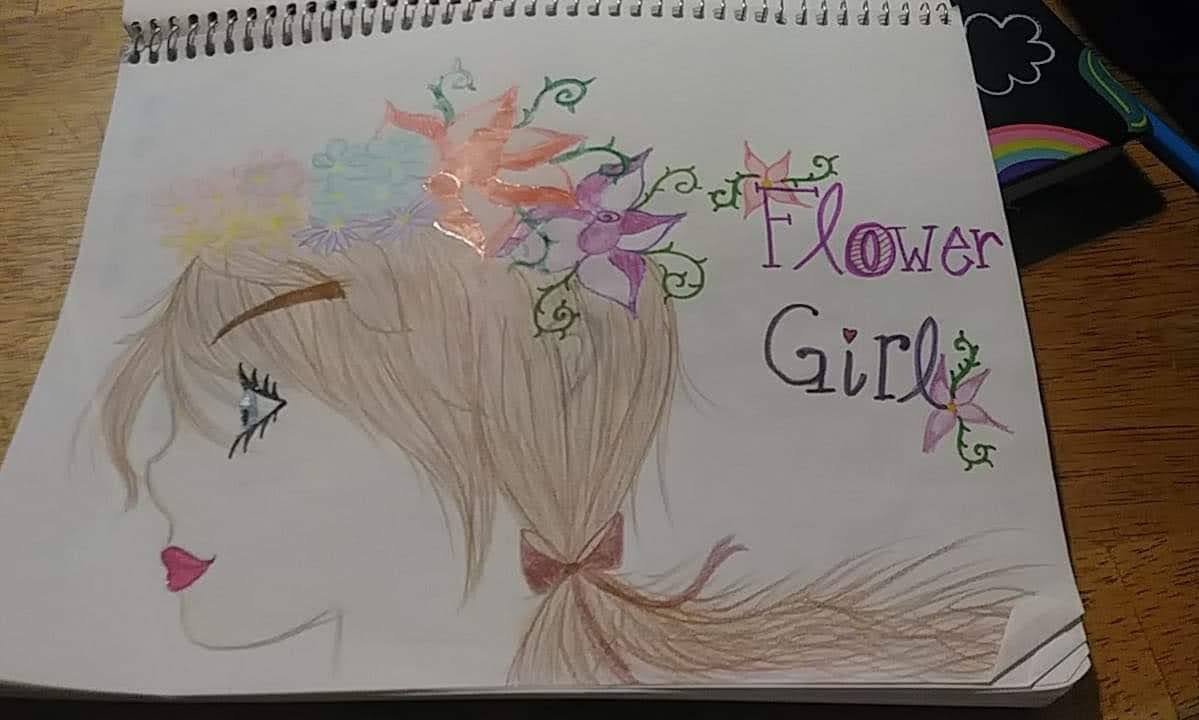In a dimly lit room, a photograph captures an open sketchpad resting on a wooden surface. The image is oriented so that the spiral binding of the sketchpad runs across the top, displaying the right side of the sketchpad sideways. Behind the sketchpad, a black cardboard book cover is visible, adorned with a colorful drawing of a rainbow and a cloud. The sketchpad features a multimedia artwork of a woman in profile, facing left. She has brown hair tied back in a ponytail, drawn with colored pencils, and her hair is embellished with numerous flowers. To the right of the drawing, the words "Flower Girl" are written in purple marker.